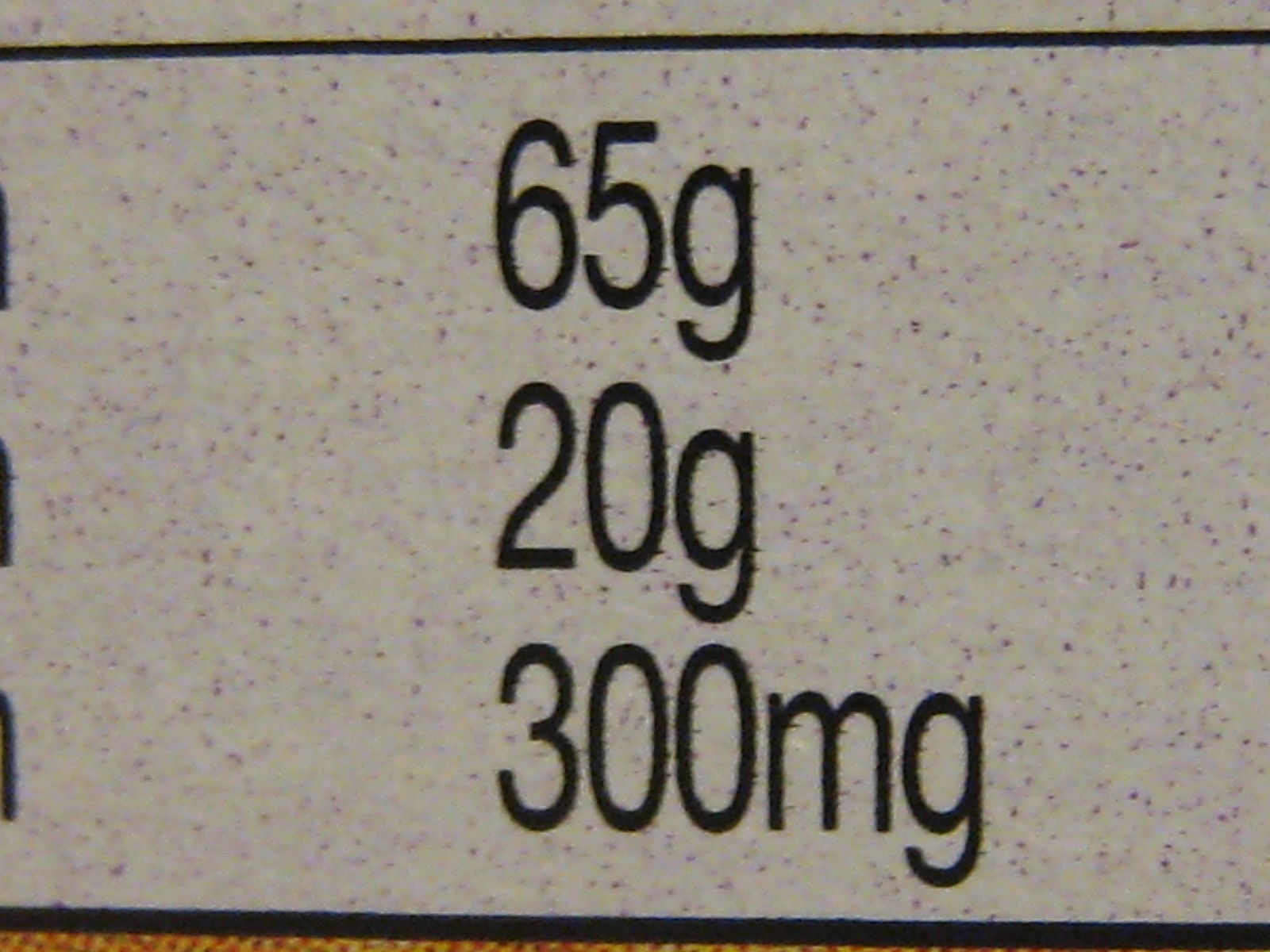This image portrays a segmented nutritional label featuring a minimalist design. The top section, set against a sparkling white background, prominently displays "65g" in bold lettering. The midsection highlights "20g" in a similar fashion, while the bottom part of the label indicates "300 milligrams." The background's white, speckled pattern adds a subtle texture to the overall visual. A distinctive black bar runs across the top of the label, contributing to its clean and organized appearance.